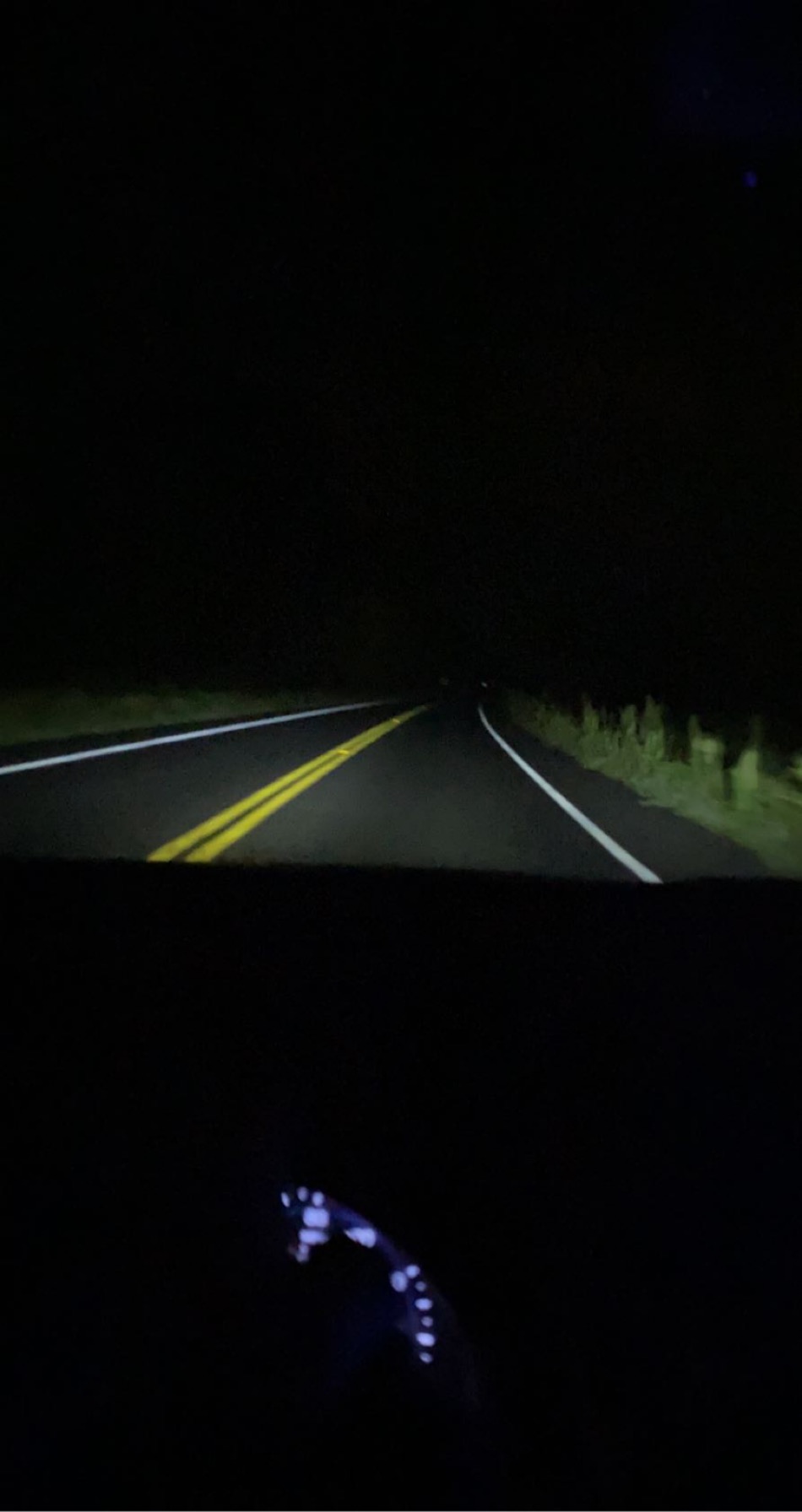The image captures the inside of a car at nighttime, with the speedometer prominently displayed. The car is traveling down a two-way street flanked by tall grass on both sides. In the distance, two bright lights—possibly the headlights of another approaching vehicle—pierce through the darkness, casting reflections on the asphalt. The night sky overhead is pitch black, and the only illumination comes from the headlights of the car in which the photo was taken, creating a stark contrast between the dark surroundings and the illuminated road ahead.